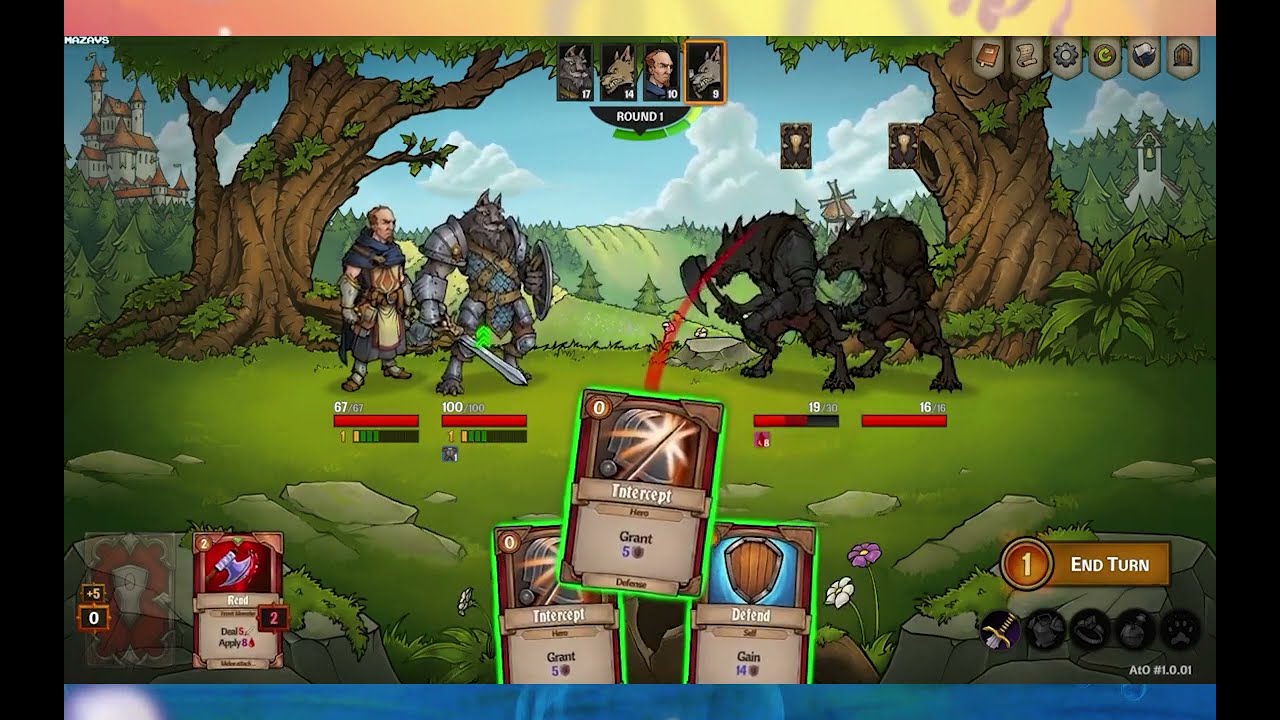This image appears to be a detailed screenshot from a medieval-themed video game, likely a digital card game, captured on a computer screen. The borders of the image have black bars on the far left and right, with a top header bar fading from reddish-yellow to yellow, and a thin blue line at the bottom footer. The central scene depicts a woodland area with green grass, trees, and two castles faintly visible in the background. On the left side, a large werewolf humanoid creature wielding a sword, wearing metal armor, and holding a shield stands in front of a human monk. On the right side, beneath another tree, are two more werewolf creatures, one with an axe marked by a red slash. 

Three cards are prominently displayed at the bottom center of the image, with legible text such as "Intercept" and "Defend." Additional game elements include an "End Turn" button circled with the number one and six circled numbers below it featuring an array of items - a sword, armor, a ring, a helmet, and a paw print. In the lower-left corner, a card portraying an axe with the number two is visible, adjacent to a semi-transparent card featuring a shield and a block labeled "+5" above a number zero. The visual style and game mechanics hint heavily at a strategy card game, mirroring elements reminiscent of "Magic: The Gathering," focused on combat and territorial conquest with fantasy medieval characters, including knights and werewolves.